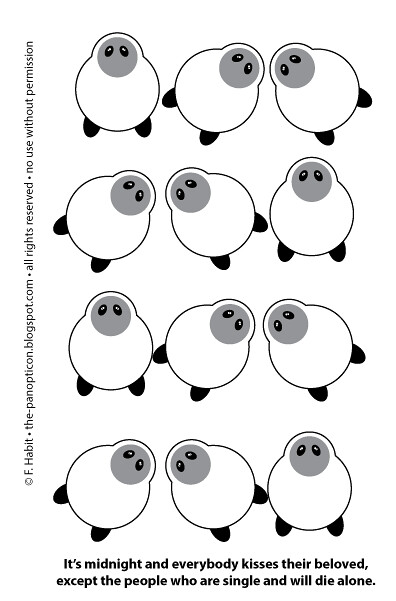The image is a detailed illustration consisting of twelve cartoon sheep organized into four rows and three columns, each sheep depicted from a top-down perspective. The sheep have white bodies with two black legs and gray faces with beady black eyes. Each row features three sheep; one faces directly forward, while the other two lean left or right. Specifically, the first and third rows have sheep facing straight up, right, and left, while the second and fourth rows mirror this arrangement. The overall style is minimalistic, using black lines and gray shapes on a white background. At the top left, text reads "f.habit.panopticon.blogspot.com All rights reserved. No use without permission." The caption below the sheep reads, "It's midnight and everybody kisses their beloved, except the people who are single and will die alone."